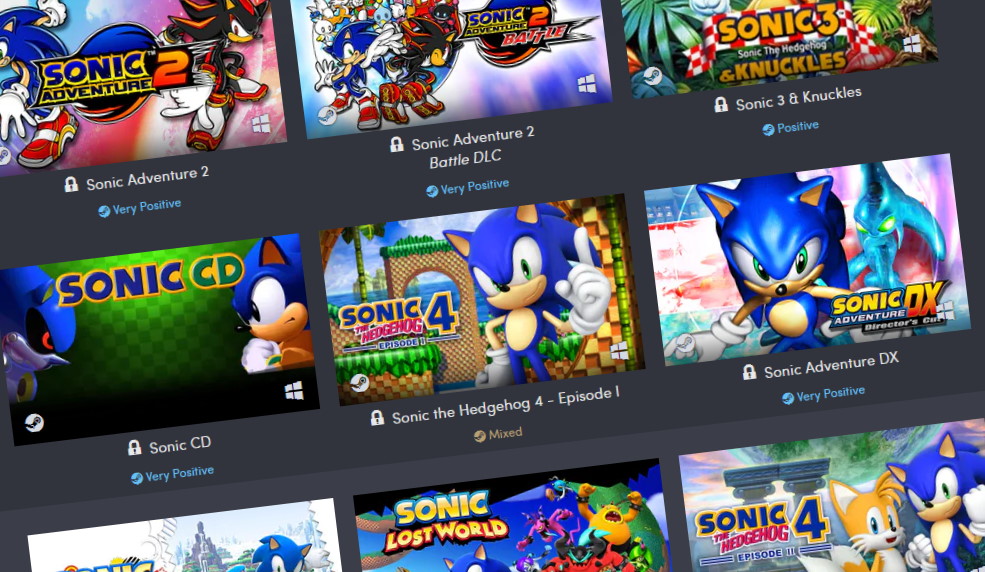This image displays a screen filled with various Sonic the Hedgehog games. The featured titles include Sonic Adventure 2, which is "very positive," although initially the game appears locked. Another game, Sonic 3 and Knuckles, also has a "very positive" rating. Sonic CD is similarly rated "very positive," but it too is locked. 

The selection notably includes Sonic the Hedgehog 4: Episode I, which has a "mixed" rating, indicating divided opinions among players. Additionally, a game titled Sonic DX is highlighted with a "very positive" rating, showing that it is well-received. 

The screen also lists other Sonic titles like Sonic Lost World and Sonic the Hedgehog 4: Episode III, but their ratings are not visible as they are partially off-screen. Overall, the display presents a diverse collection of Sonic games, showcasing a range of user ratings and availability statuses.